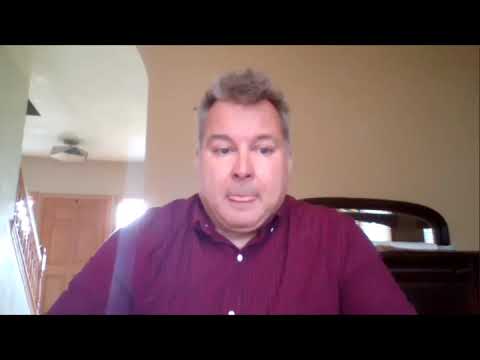In the image, a rotund man with brown hair streaked with gray is seen facing the camera, seemingly in mid-conversation during a virtual meeting on a platform like Zoom or Google Meet. He is wearing a maroon button-up collared shirt and has his tongue between his lips, as if he's wetting them or concentrating. The backdrop reveals he is in a domestic setting, with a beige wall behind him and an arched entryway leading to another room. This room features a banister railing, a door, and a ceiling light. On his left side, a dresser topped with a mirror and something white is visible. The image is bordered by thick black bands at the top and bottom, adding a frame to the scene.